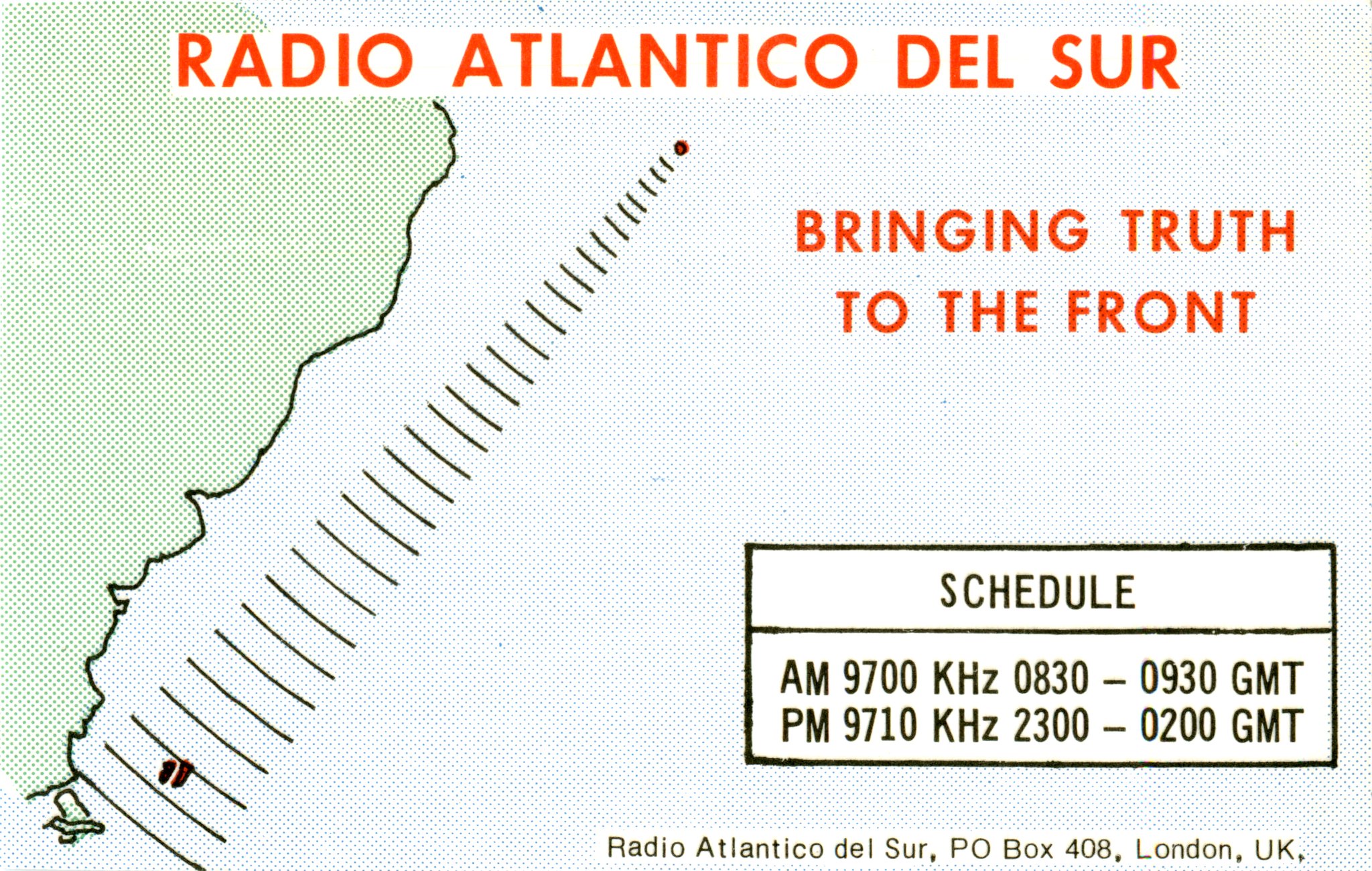The image is an informative page featuring a partial map of the UK, shaded in light green. At the top, in red lettering, it reads "Radio Atlantico del Sur." Below this, a slogan in a similar reddish-orange color declares, "Bringing truth to the front." The map displays a red dot beneath the word "Atlantico," with black wave-like lines emanating from it, symbolizing radio signals. In the bottom right corner, there's a rectangular legend detailing a radio broadcast schedule: "AM 9700 KHz 0830-0930 GMT" and "PM 9710 KHz 2300-0200 GMT." Additionally, the corner provides a contact address: "Radio Atlantico del Sur, PO Box 408, London, UK."